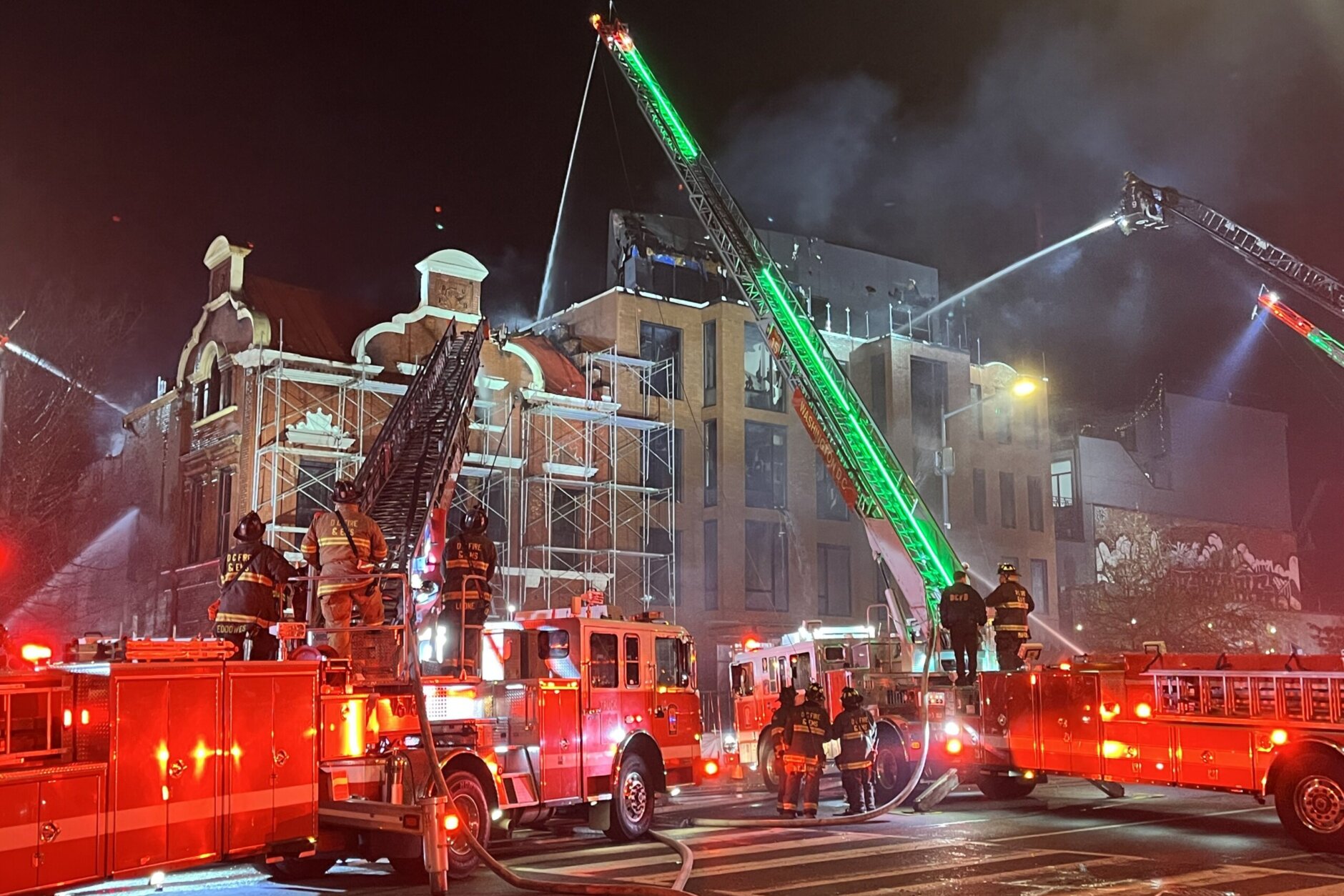This photograph captures a nighttime scene of multiple fire engines and firefighters combating a blaze at a four-story city building covered in silver scaffolding. The well-lit setting primarily shows two fully visible fire engines, one with a black ladder and the other with a green ladder, positioned on a dark grey asphalt road marked by white crosswalk lines. The building, likely an office or government structure with a brick front, is partially obscured by smoke and water vapor. At least two additional fire engines are evidenced by multiple ladders extending into the top right corner of the image. A central crane, the tallest and illuminated by a green neon light, sprays water onto the building, while other cranes in the scene, including two black ones, assist in the operation. Approximately ten firefighters are actively monitoring the situation from the trucks and sidewalk, collectively ensuring the fire is under control.